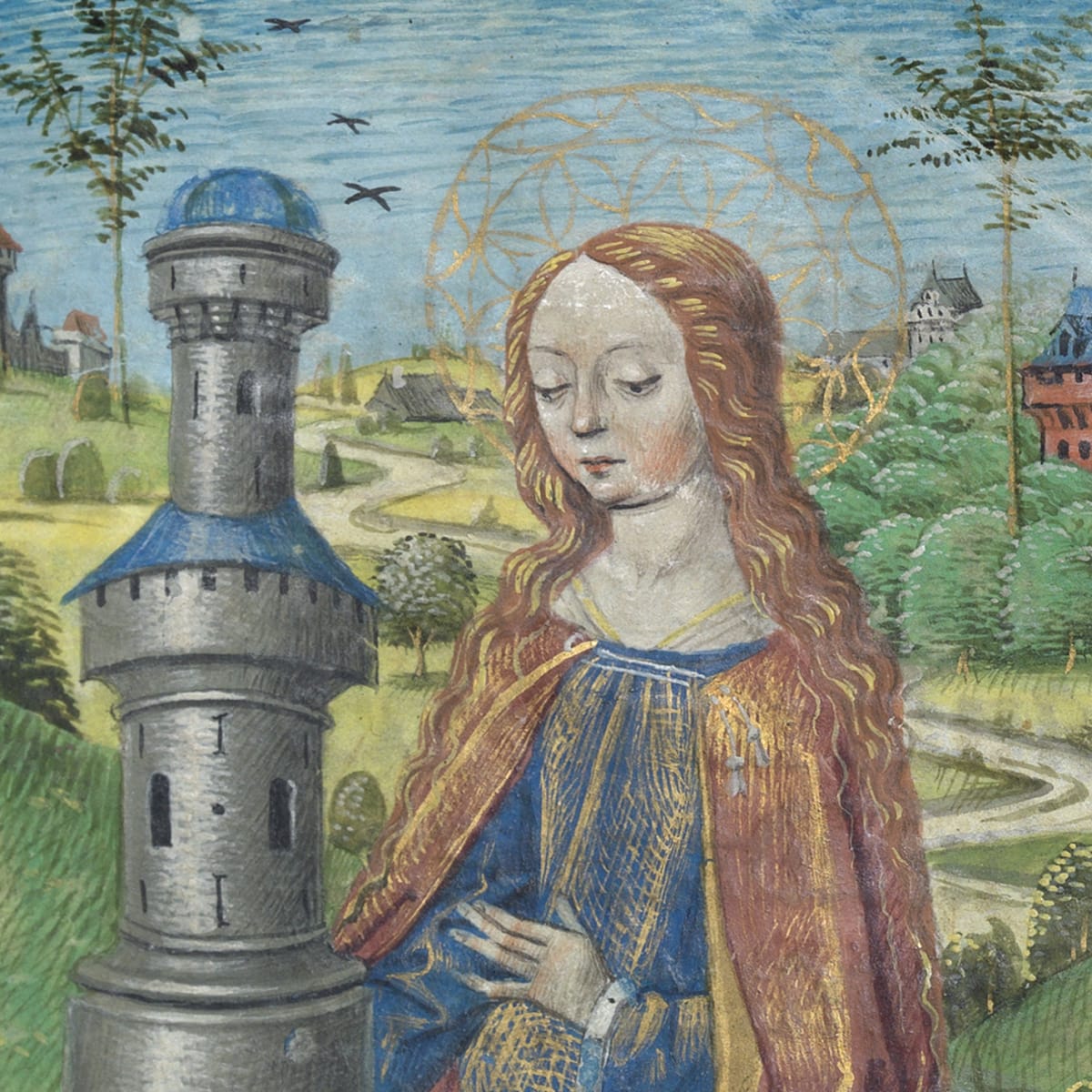This image is a detailed painting set in an earlier time period, likely medieval, Victorian, or Renaissance. The sky, textured with hues of blue and gray-white, hosts three birds in flight. Dominating the foreground is a woman dressed in an ornate blue gown with gold accents running down the center. Over this, she wears a gold robe that transitions into hues of orange, red, and yellow. Her long, blonde hair cascades down her torso, giving her a Rapunzel-like appearance. She is adorned with gold necklaces and a bracelet, while a crown or an aura-like head cover, resembling a fancy net, adds a saintly aura to her figure. She stands beside a small castle or model of a castle, making it appear as if she's in a fairy tale setting. Flanking her are trees on both the left and right, with additional green shrubbery and bushes in the foreground. In the background, a red brick building is visible, with a road that winds its way to the rear of the scene, completing this richly detailed and vibrant painting.